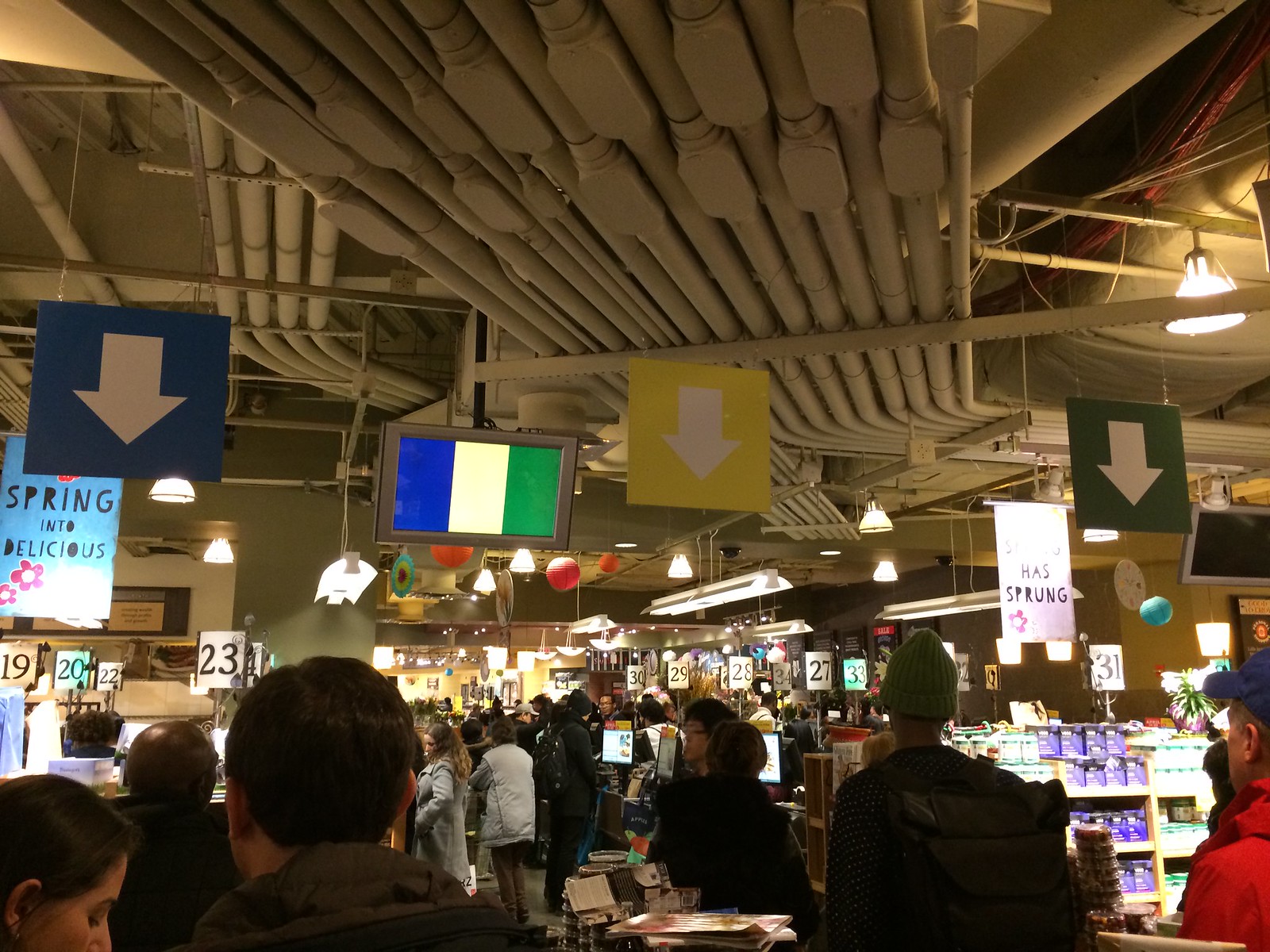This image captures the bustling interior of a large, warehouse-like grocery store with high, unfinished industrial ceilings showcasing exposed pipework, ducting, and lighting fixtures. The store is notably crowded, with over twenty customers dressed in dark, winter outdoor clothing, some in woolly hats and large jackets, indicating cold weather outside. In the foreground, a group of people is gathered, looking deeper into the store.

Several colorful signs with white arrows pointing downwards hang from the ceiling, directing customer flow towards various checkout lines. Among them, notable signs include a prominent blue sign with the text "Spring into Delicious," adorned with pink flowers, and a large yellow sign with a white arrow. Signs indicate checkout numbers such as 19, 20, 22, 23, 27, 28, 29, and 30. There is also a country flag visible near the center, though its specific origin is indeterminate. Throughout the scene, advertising signs and organizational signage, some in blue, yellow, and green, enhance the commercial atmosphere, creating a palpable sense of order amidst the chaotic hustle and bustle of the grocery store environment.